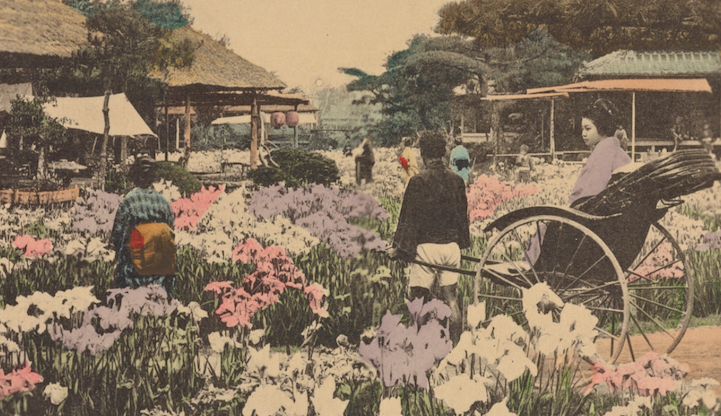The image appears to be an intricately colored, old-fashioned print, resembling a traditional cartoon rather than a realistic photo. The scene is richly detailed, featuring a vibrant field in the foreground filled with pink, white, and purple flowers interspersed with tall grass, and surrounded by various shades of green trees in the background. On the left side of the image, a woman dressed in a dark blue kimono stands near a series of small, thatched-roof structures supported by four pillars, open on all sides, with paper lanterns hanging from the eaves. In the center, an array of colorful flowers blooms, adding splashes of color to the scene. On the right side, a woman wearing a colorized purple kimono sits in a black rickshaw with two large wheels, being pulled by a man dressed in a black outfit with short white pants. Additional background details reveal a few figures milling about this tranquil, traditional Japanese setting.